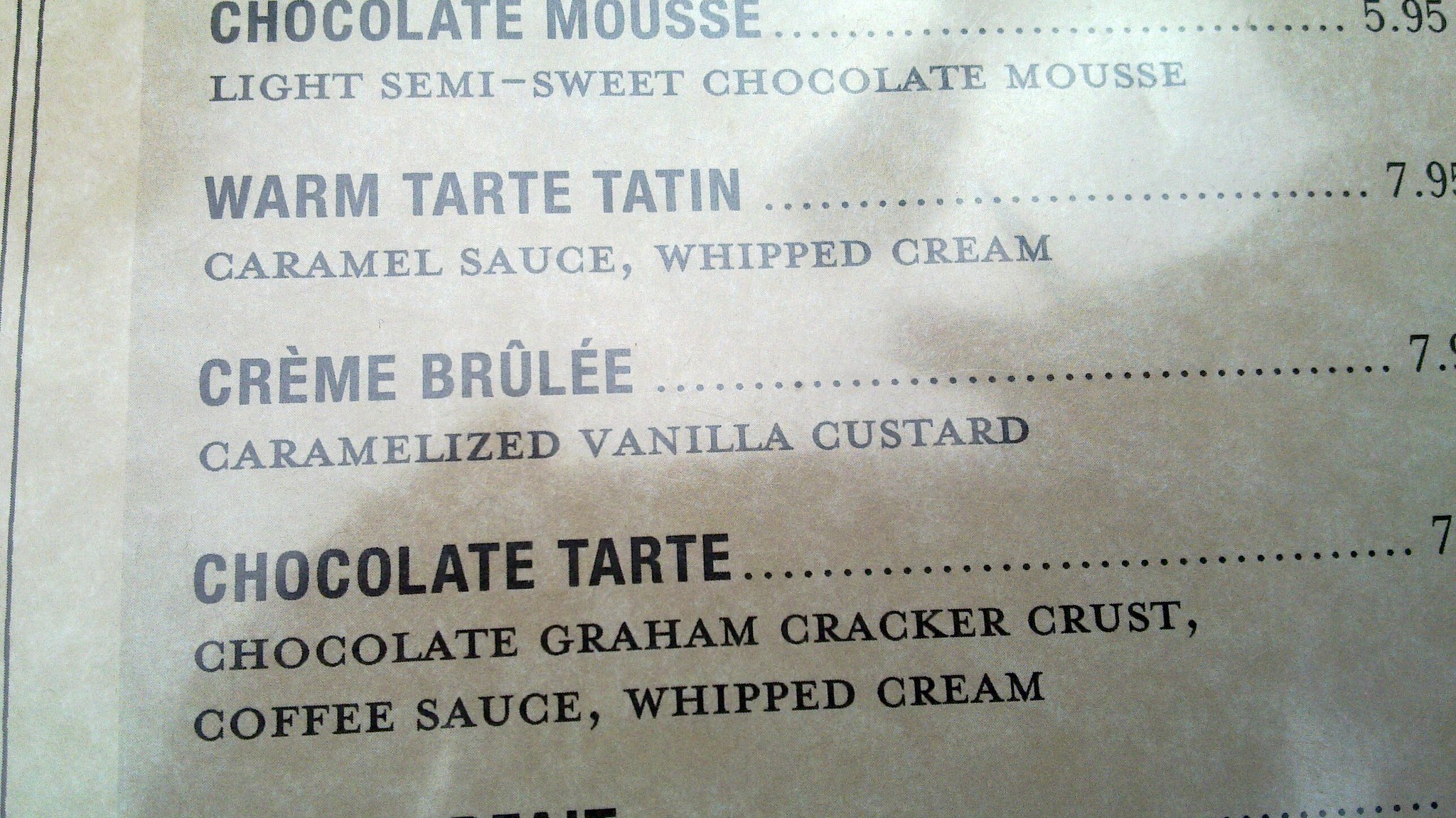This image captures a closely-cropped excerpt from a dessert menu, slightly askew and featuring some obscured lettering. The menu, appearing off-white, is either reflecting something dark behind it or has a noticeable stain. Despite the angle and cropping, several dessert items and their prices and descriptions are visible. 

In bold, black lettering, the menu lists "Chocolate Mousse," "Warm Tart Tatin," "Crème Brûlée," and "Chocolate Tart." The price for Chocolate Mousse is clearly marked at $5.95, while the other desserts' prices are partially visible, each starting at $7—specifically, the Warm Tart Tatin appears to cost $7.95. Underneath each dessert name, detailed descriptions are provided: the Chocolate Mousse is described as a "light semi-sweet chocolate mousse"; the Warm Tart Tatin includes "caramel sauce and whipped cream"; the Crème Brûlée is a "caramelized vanilla custard"; and the Chocolate Tart features a "chocolate graham cracker crust, coffee sauce, and whipped cream." The image, though imperfect, gives a clear sense of the tempting offerings available.